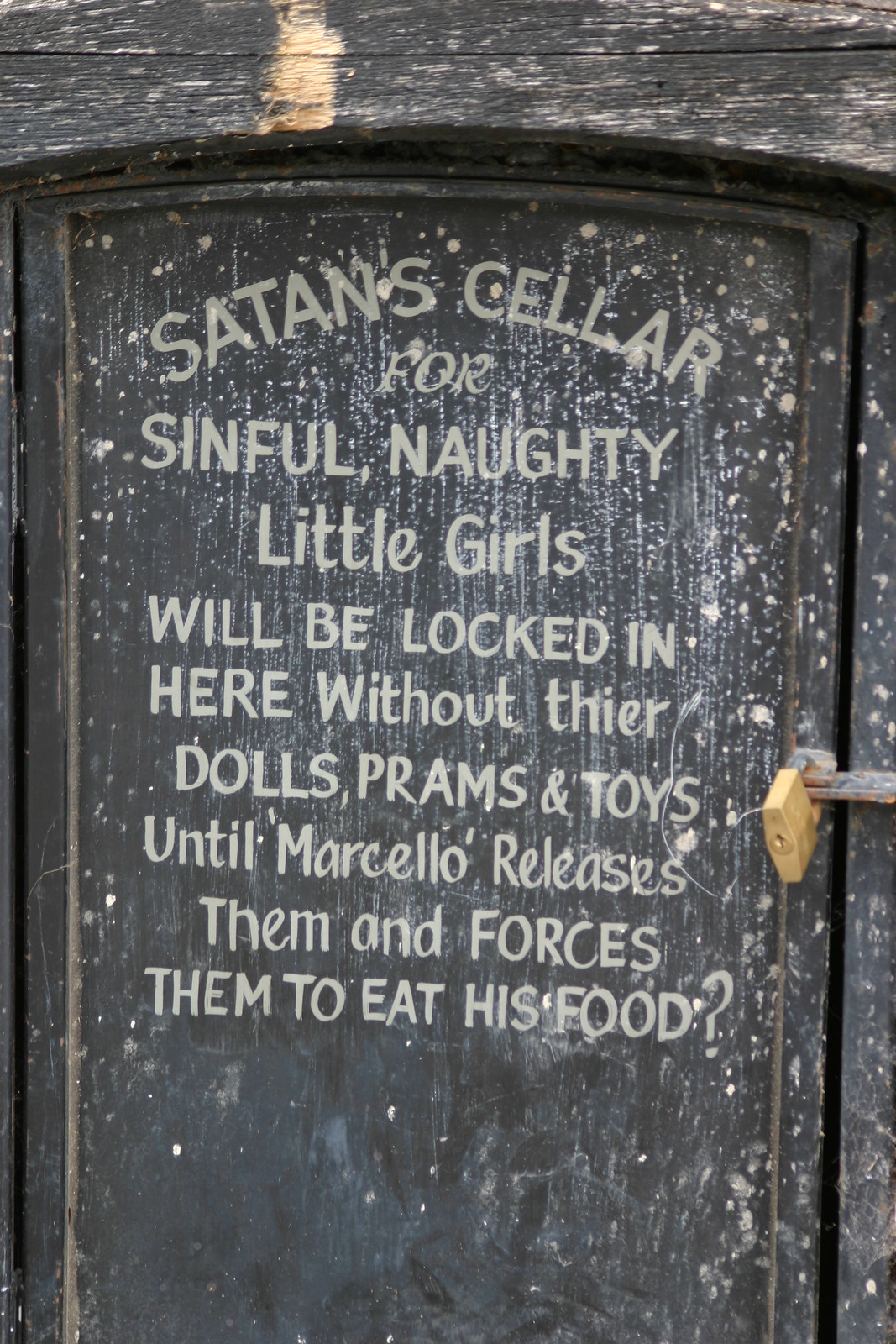The image features an aged wooden cellar door located outdoors, evidenced by the weathered wood. The door, shorter than typical doors, is secured with a new bronze padlock that has a gold base and a silver hook positioned on the right side. The entire construction, including the top cover, is made of wood, and the door is marred with paint splashes, grime, and dirt residues. At the top of the door, centered, there is a handwritten message in white paint, arranged in an arc-shaped direction. The message reads: "Satan's cellar for sinful, naughty little girls will be locked in here without their dolls, prams, toys until Marcello releases them and forces them to eat his food." Despite the paint and dirt splatters covering parts of the door, the unsettling text remains fully readable.